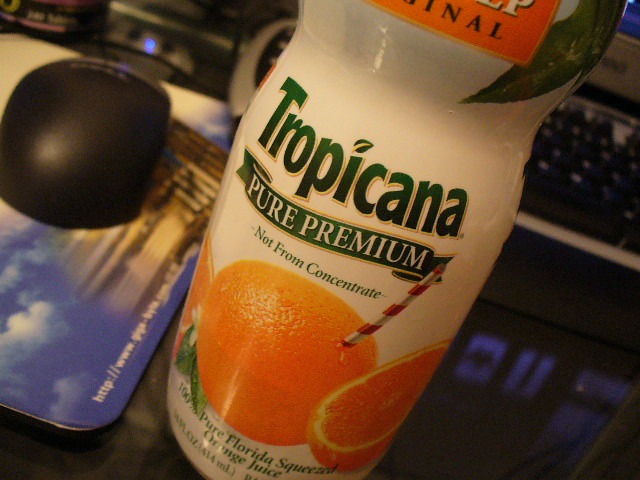The image features a white plastic bottle with an orange label at the top, displaying the word "anal." Below the orange label, green text spells out "Tropicana" with a distinctive leaf adorning the letter "I." Under the brand name, the phrase "Pure Premium" is printed, followed by "Not from Concentrate" below it, all in clear, bold letters. The design is completed with an illustration of an orange impaled by a straw, suggesting the concept of fresh orange juice, although this depiction is noted to be unrealistic as one cannot drink directly from an orange with a straw.